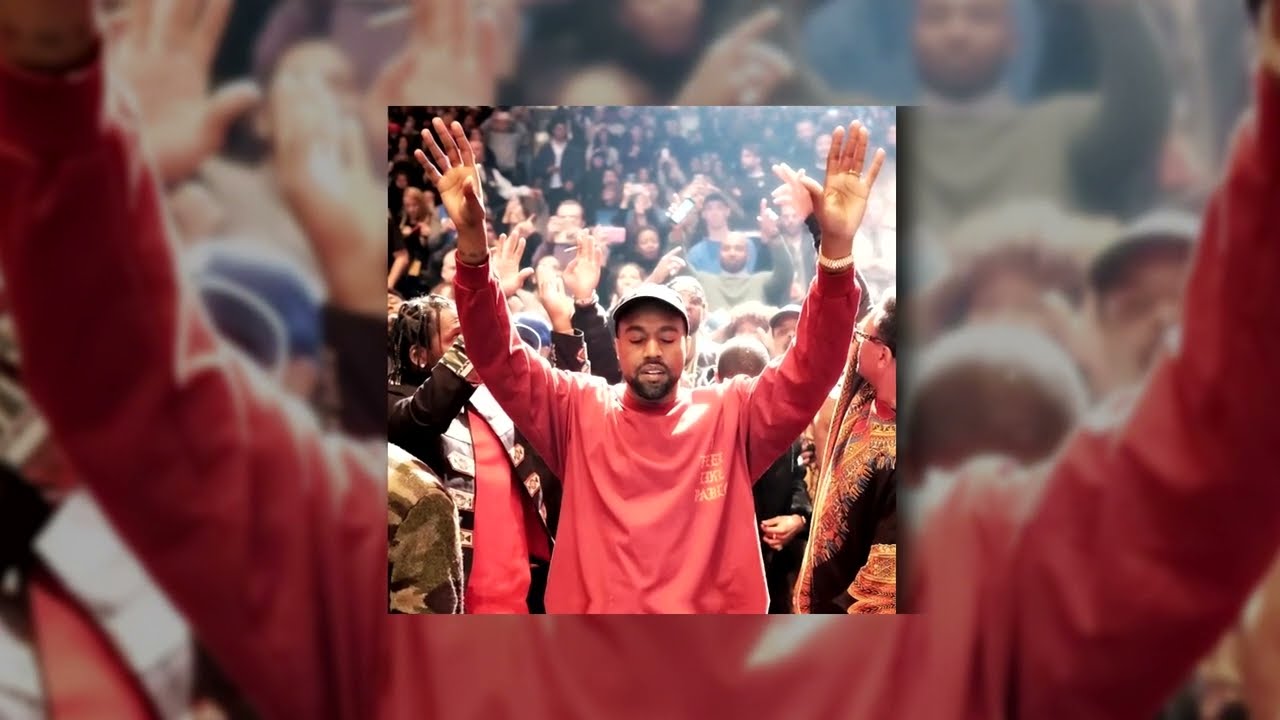In the center of the image, a man reminiscent of Kanye West stands with both arms raised in a pose suggestive of praise, his eyes closed. He sports a red long-sleeve shirt with yellow text on the chest area and a grayish baseball cap, along with a black goatee. Behind him, a large, diverse crowd mirrors his gesture, many with their arms similarly raised, likely indicating a collective moment of worship or celebration. To his left, a man with dreadlocks in a similar red sweatshirt and a black jacket stands, while on the far left, a white man wears a black-and-gold African tribal shirt. The background around this central image is a blurred and faded zoom-in of the same picture, creating a frame that extends to the left, right, top, and bottom. Light emanates from the upper right corner, casting a glow that highlights the heads of the crowd, enhancing the sense of depth and focus on the man and the collective crowd behind him.